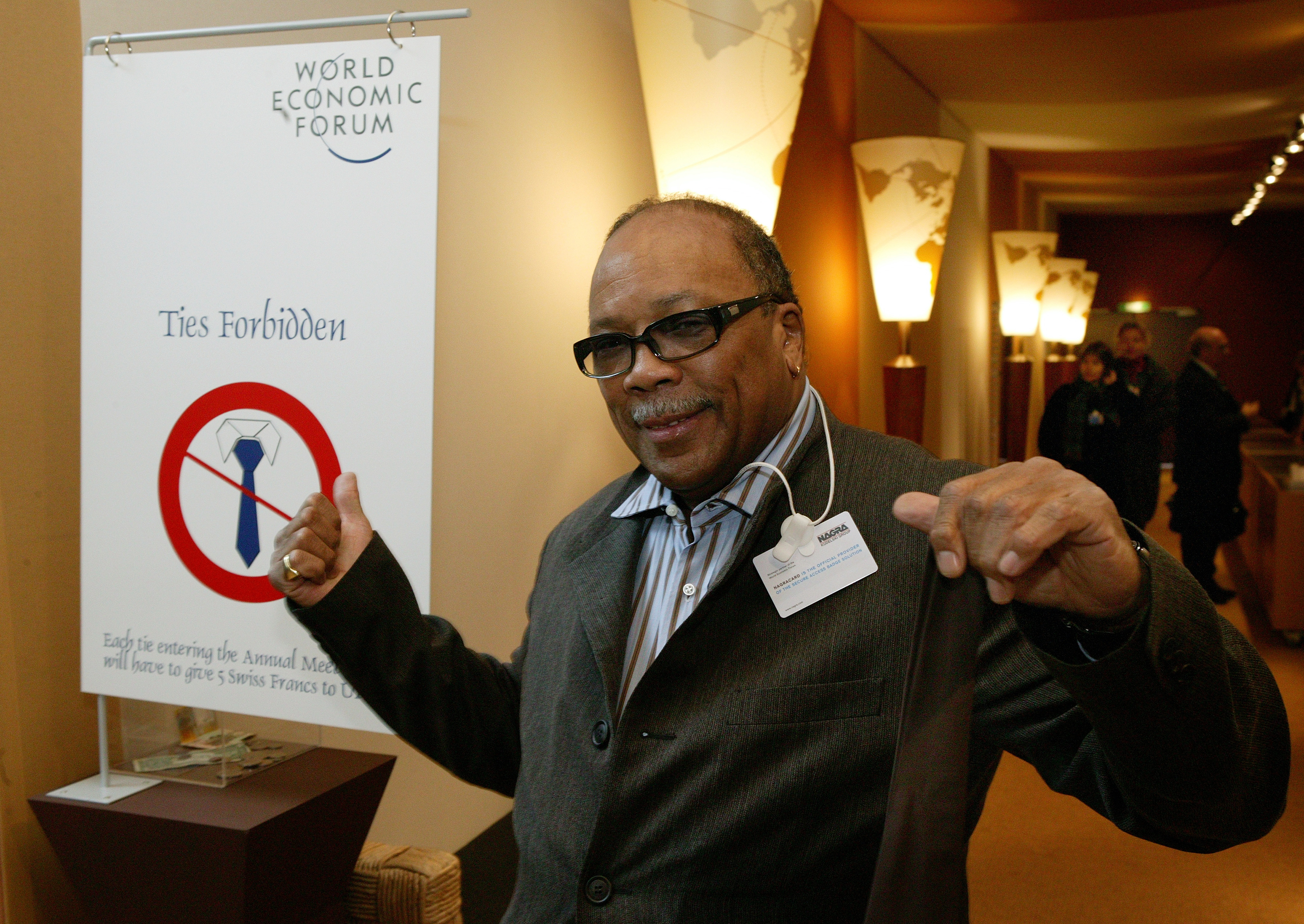The photograph captures Quincy Jones, centered in the image with both hands slightly raised and semi-closed, as if he's about to dance. He is wearing a dark gray suit jacket, buttoned up, paired with a striped shirt that seems to be either light blue or white with red and blue stripes. Jones sports black rimmed glasses, has short dark brown hair, and a distinct gray mustache.

To his left, a sign prominently reads "World Economic Forum" at the top, followed by "Ties forbidden." The sign humorously features an image of a crossed-out tie and notes that any tie entering the annual meeting incurs a fee of five Swiss francs. In the background, slightly blurred, are several other people dressed in dark clothing, standing in a hallway. A series of lights behind them and leading up to Quincy resemble cylindrical globes, adding an interesting element to the setting, which appears to be a lobby or conference area. Quincy, notably tieless, seems well-prepared for the event's quirky dress code.